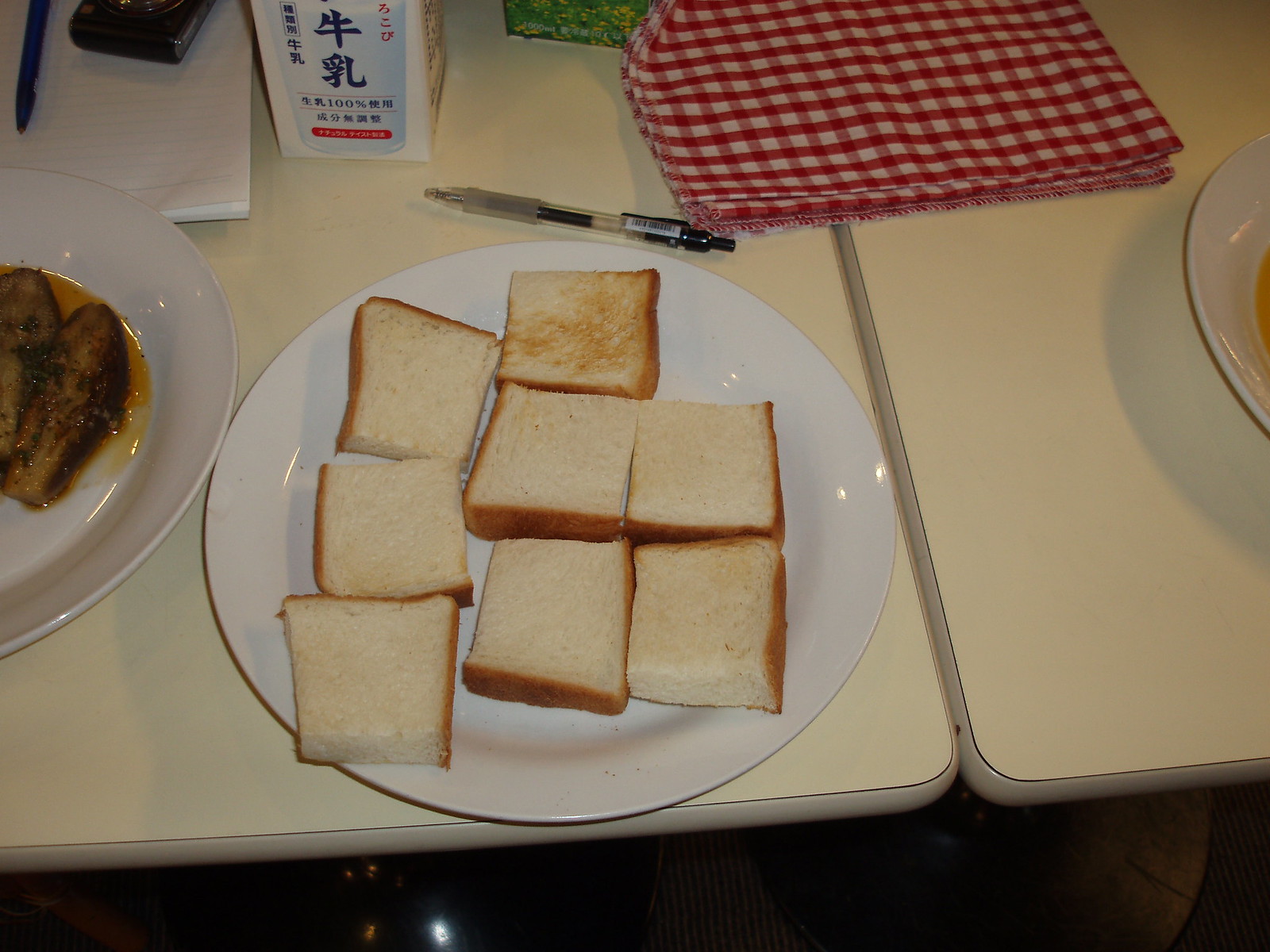The image depicts a white dinner plate with a gold rim, holding six to seven small square pieces of white bread, most of which appear untoasted except for one with a slight golden brown hue. The plate is placed on what seems to be two adjoining white tables, possibly made of plastic or a hard laminate. We can see partial views of the plates to the left and right of the central bread plate: the left plate contains what might be fried food or meat with an orange or yellow-brown sauce, while the plate on the right, farther away, mostly shows just a gold-rimmed edge. A folded red napkin spans the junction of the two tables. There is also a black push-to-click ballpoint pen lying above the bread plate and a white box labeled in Japanese characters nearby, displaying "100%" prominently. Additional items include a hint of a red and white checked cloth in the background, along with what appears to be some scattered papers and possibly a phone or remote control.